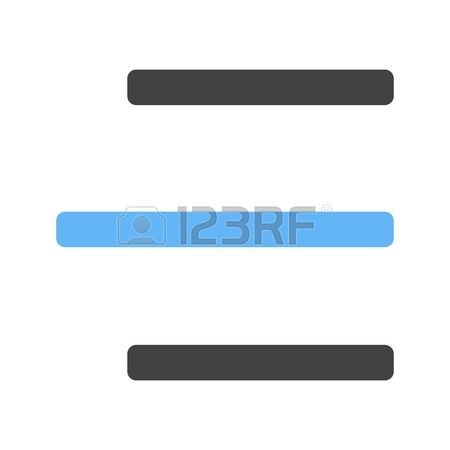The image features a minimalist design on a white background, consisting of three horizontal bars with rounded corners. The top and bottom bars are thin and black, extending across the width of the image. Positioned centrally between them is a slightly longer horizontal blue bar. Overlaid on the blue bar is an icon representing a person, depicted by a gray circle as the head and a separated torso, all encircled by a thin gray emblem. The bar also contains the numbers "1, 2, 3" and the letters "RF" in a light gray or possibly purple hue.